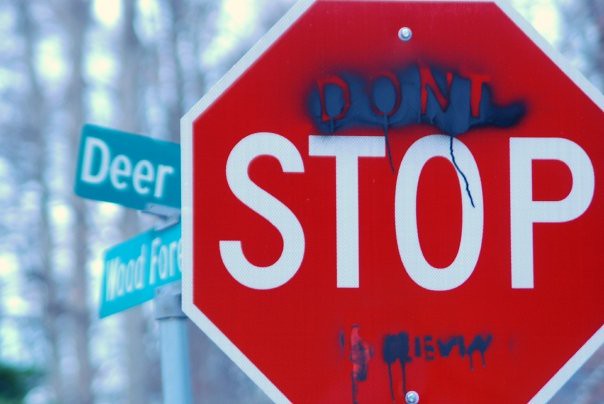This outdoor picture features a prominent stop sign at the forefront. The stop sign is classic red with a white border and the word "STOP" in white letters. However, it has been defaced with graffiti, including a blue stencil design that spans the letters "O" and "T," with some blue paint dripping through the "O" and additional spots of blue at the bottom. Close to this stop sign, to the left, stands a green street sign supported by a steel pole. The top portion of this sign reads "DEER" and the bottom part appears to say "WOOD FOREST." The letters are slightly obscured but legible. In the background, the image is blurred, with hints of tall trees and sunlight filtering through, giving a serene yet somewhat indistinct natural setting.